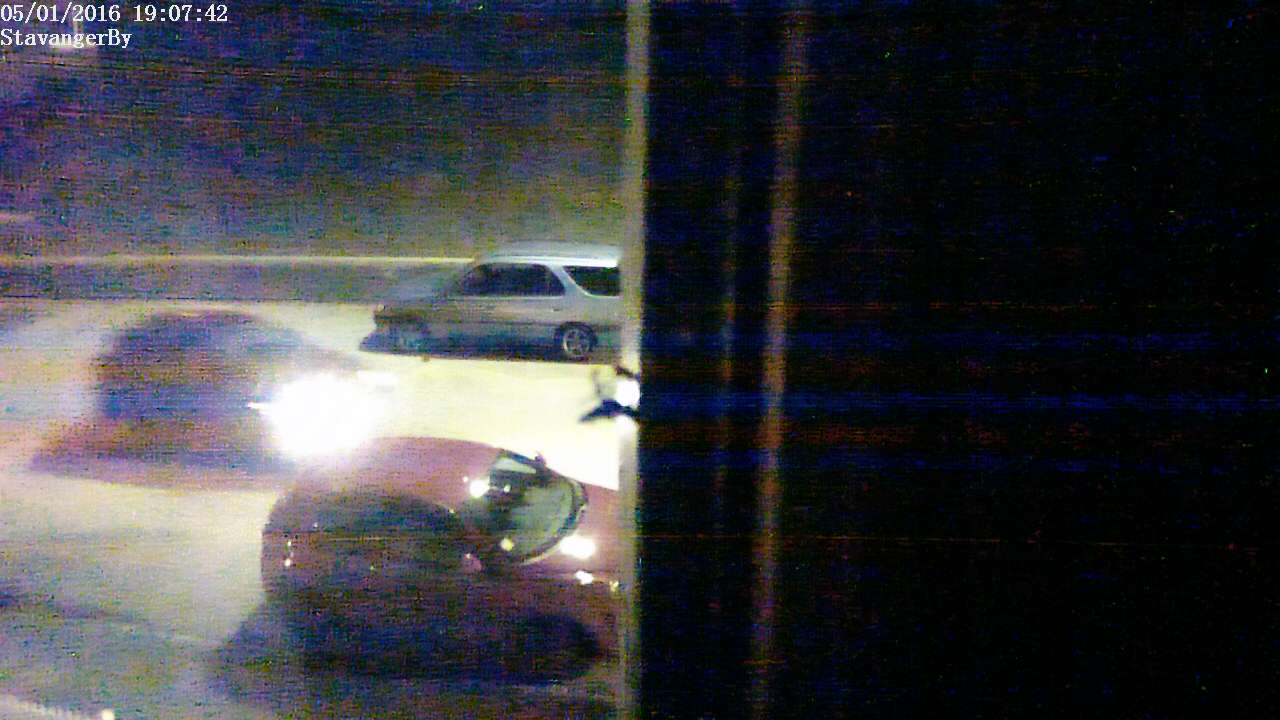A photograph captured from an indoor vantage point, possibly through a window or doorway, features a juxtaposition of darkness and artificial illumination. On the right side of the image, a wooden panel partially obscures the view, casting a shadow that contrasts starkly with the illuminated left side. The left side reveals a busy freeway with vehicles traveling in both directions. Prominently, a red sedan is moving from left to right, followed by another car whose headlights create a burst of light, partially obscuring the scene. In the opposite direction, a gray SUV with tinted windows traverses the freeway, adding a sense of motion and dynamic contrast to the composition.